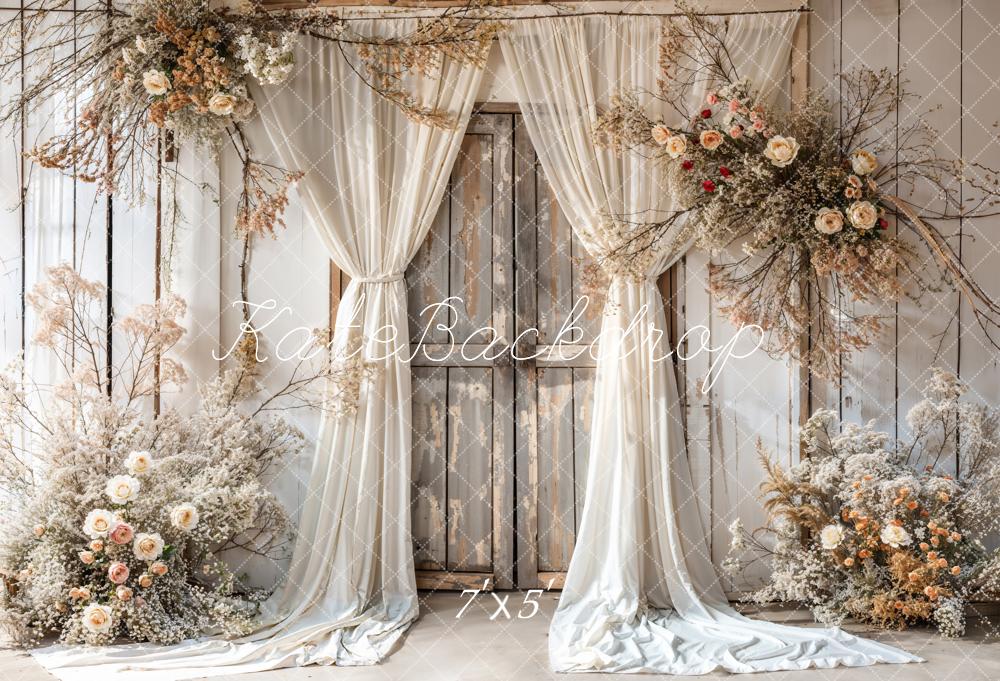The image showcases a boho chic styled backdrop designed to resemble the backside of a small wooden storage shed or barn. The side of the building is made from vertical wooden boards with two central, distressed gray barn doors. These doors are artistically adorned with translucent, white silk curtains, gathered and tied in the middle, creating an elegant entranceway. Placed around the backdrop are vibrant bouquets of flowers in pink, red, orange, white, and yellow, positioned in the top left, top right, bottom left, and bottom right corners, adding a splash of color and charm. The backdrop, which is intended for photography purposes, includes the text "Kate backdrop 7x5" in the center. The entire image is overlaid with crisscross patterns to prevent copyright infringement.